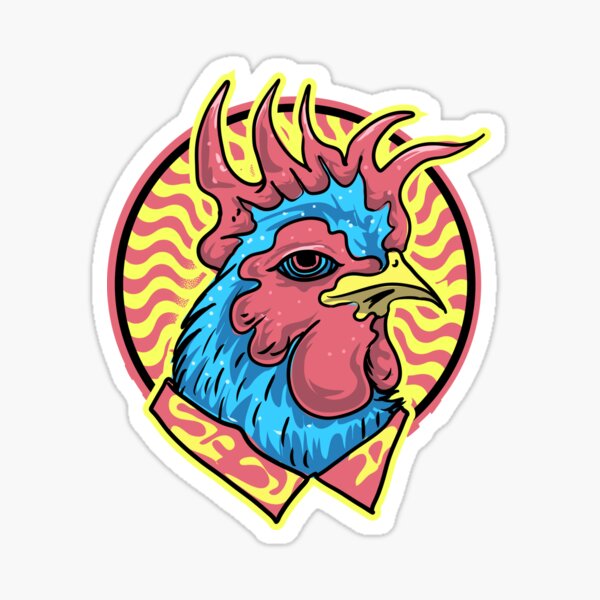This photograph captures a graphic-like sticker or magnet featuring an abstract representation of a rooster. The image is surrounded by a white border, followed by a red one, encircling the rooster's head. The bird's visage is framed by squiggly red and yellow stripes within a pink and black border. The rooster's head is predominantly blue with detailed, multi-colored eyes—showcasing swirls and half-moon shapes in shades of pink, blue, and dark blue with a black center. The eyes also include white speckles. A striking red, flame-like crown not only adorns the top of its head but also gives it a wild, untamed appearance. The rooster has a yellow beak and appears to be wearing a collar that mirrors the pink and yellow patterns in its surroundings, hinting at a shirt. The overall design combines vibrant colors and chaotic patterns to create a surreal, eye-catching piece.